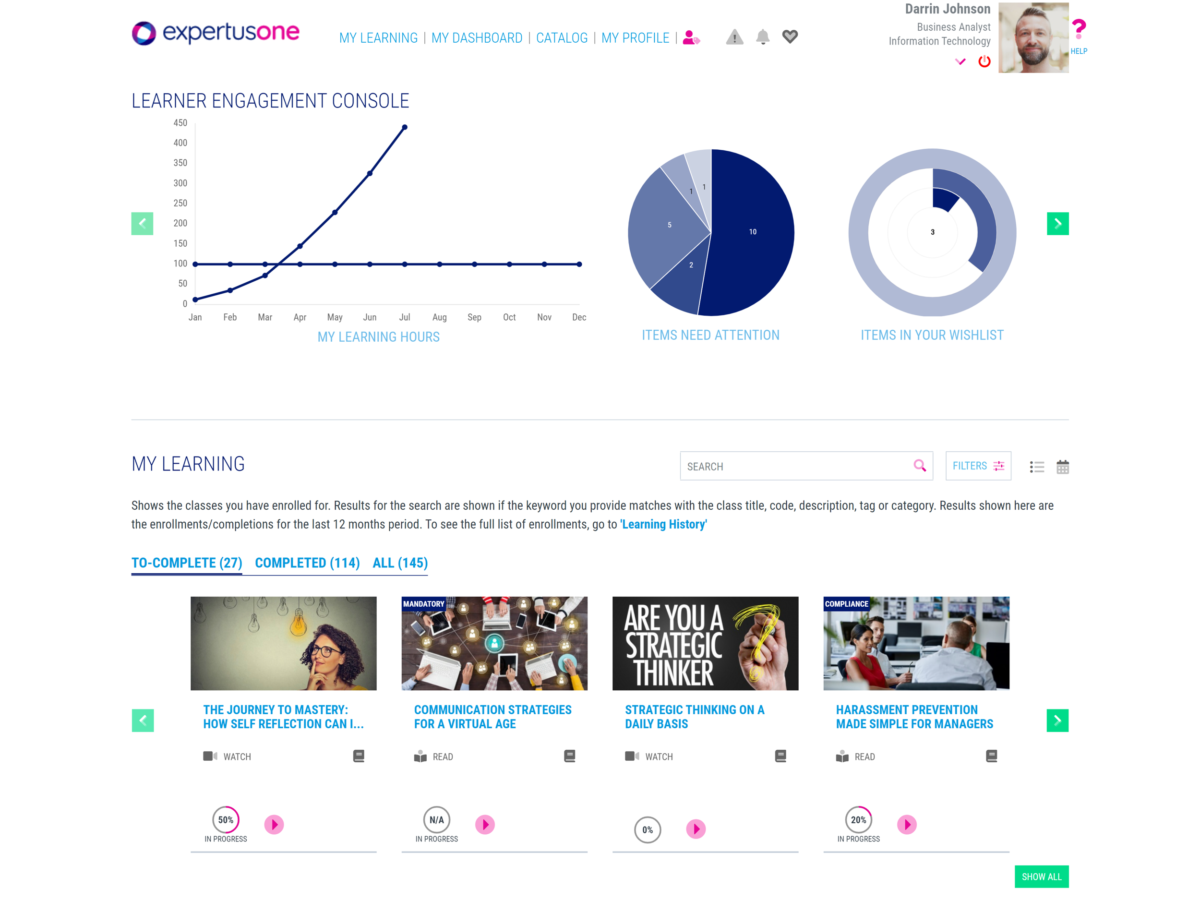Here is a detailed and cleaned-up caption for the image:

---

**Screenshot Description: Expertus1 Learning Management Platform**

The screenshot showcases the landing page of the Expertus1 learning management website, which is designed to enhance learner engagement. Central to the interface is a "Learner Engagement Console" graph, accompanied by two adjacent pie charts. These visualizations likely provide insights into user engagement metrics.

An organized section titled "My Learning" is displayed prominently. This section is divided into three tabs:
1. **To Complete**: Lists 27 items pending completion.
2. **Completed**: Displays 114 items that users have already finished.
3. **All Items**: Summarizes a total of 145 items across both completed and pending tasks.

Below this section are four thumbnail images acting as links to different courses or tasks. These multimedia learning materials include both video and text-based formats, indicated by play buttons and text icons.

The overall color scheme features a clean, white background with varying shades of blue—ranging from dark to light—and accents of bright pink. The text on the page predominantly uses these blue hues, enhancing readability and visual appeal. The bright pink is also used for the play buttons of the courses at the bottom, creating a cohesive and vibrant look.

In the upper right-hand corner, there is a professional headshot presumably of an employee, Darren Johnson, titled as "Business Analyst, Information Technology." His profile likely provides quick access to user or account settings.

**Visual Style:**
- Background: White
- Primary Colors: Shades of blue (dark to light)
- Accent Color: Bright pink
- Text: Various shades of blue

This detailed layout aims to provide an intuitive and engaging user experience, facilitating seamless navigation and interaction with the platform's learning resources.